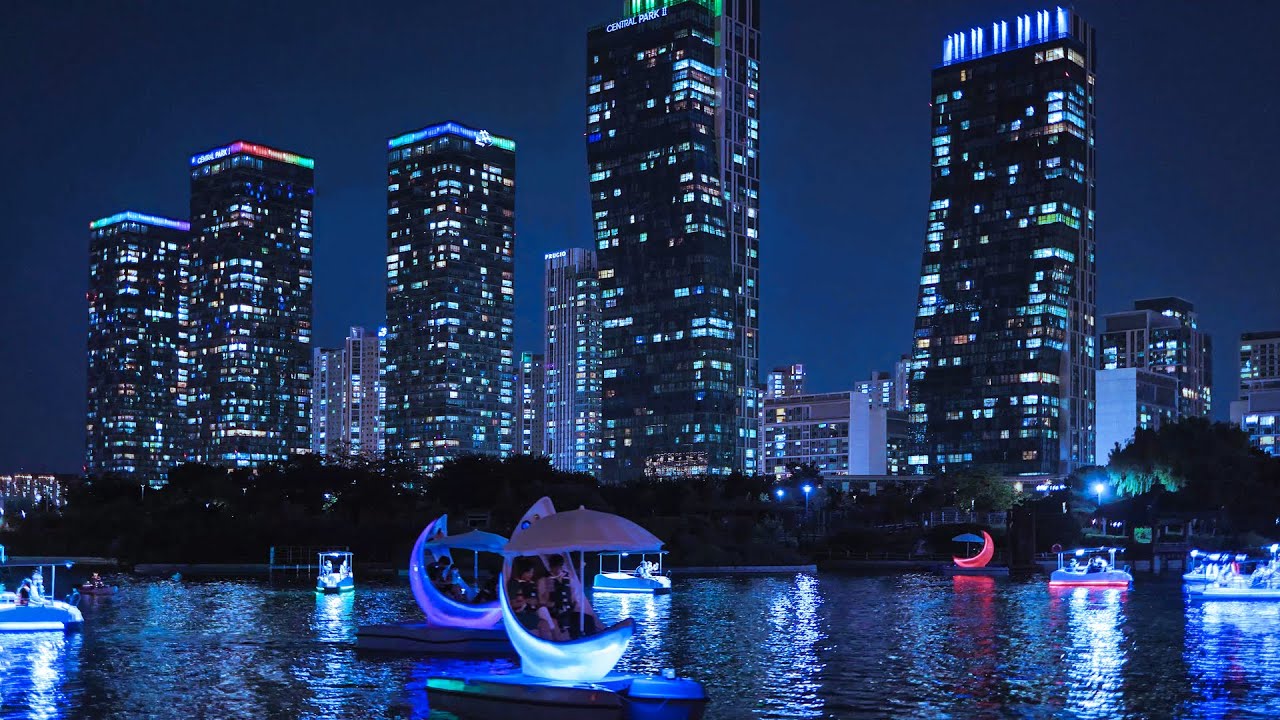This captivating nighttime photograph captures an urban cityscape with a strikingly vibrant skyline. The image showcases numerous tall, narrow skyscrapers, each approximately 25 stories high, brilliantly illuminated with multicolored lights at their summits—ranging from red, blue, green, and yellow to orange and fluorescent hues. The windows of these steel high-rises emit a mix of colored glows, suggesting activity within the buildings.

In the foreground, a serene body of water, possibly a lake or river, mirrors the dazzling city lights, enhancing the nighttime ambiance. On this water, several neon-lit paddle boats drift gracefully. These boats, each resembling a crescent moon with bright LED illumination, come in a variety of colors, including purple, green, pink, and blue, casting a magical glow onto the water below. Each boat is equipped with a large beach umbrella and a pontoon base, providing a cozy seating area for occupants. The scene showcases paddle boaters, some appearing as families with children, enjoying the serene night.

Interspersed between the tall buildings at the city's edge, a line of trees hints at a nearby park, adding a touch of nature to this vibrant urban oasis. The sky, a deep midnight blue, completes the enchanting scene, making it both a stunning and serene nighttime vista.